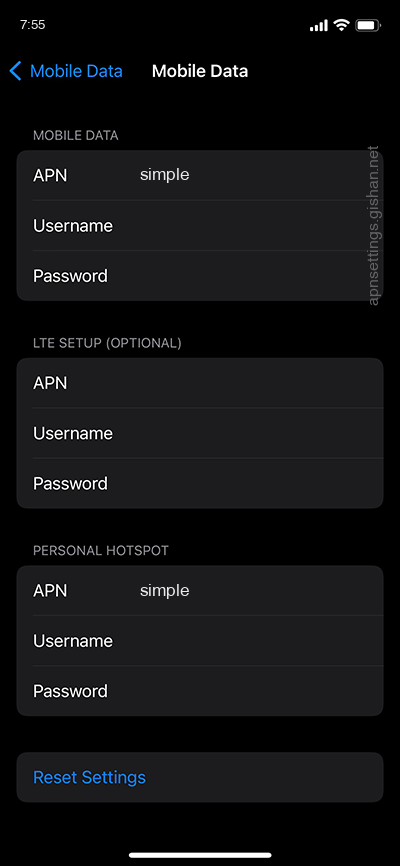This screen capture from an iPhone, displayed in dark mode, features a typical interface with ribbons at both the top and bottom of the screen. At the top, there are two tabs labeled "Mobile Data"; the tab on the left is highlighted in blue, while the one on the right remains white. 

Immediately below, we see various configuration fields: the first section, under the highlighted "Mobile Data" tab, has the text "APN" in bold capital letters, followed by fields for "Username" and "Password."

Next, there is a header labeled "LTE Setup Options," which includes fields for "APN," "Username," and "Password," all in capital letters for "APN" and capitalized first letters for the other words. 

Further down, there is a section titled "Personal Hotspot," which also features fields for "APN," "Username," and "Password," maintaining the same capitalization format as mentioned above.

At the very bottom of the screen, there's an option to "Reset Settings," prominently displayed in blue font.

The entire screen maintains a monochromatic theme with black backgrounds and white font, except for the blue highlights indicating active selections and interactive options (the "Mobile Data" tab and "Reset Settings"). There are no overlays or additional visual elements. This screen appears to be dedicated to configuring various mobile data settings on the iPhone.